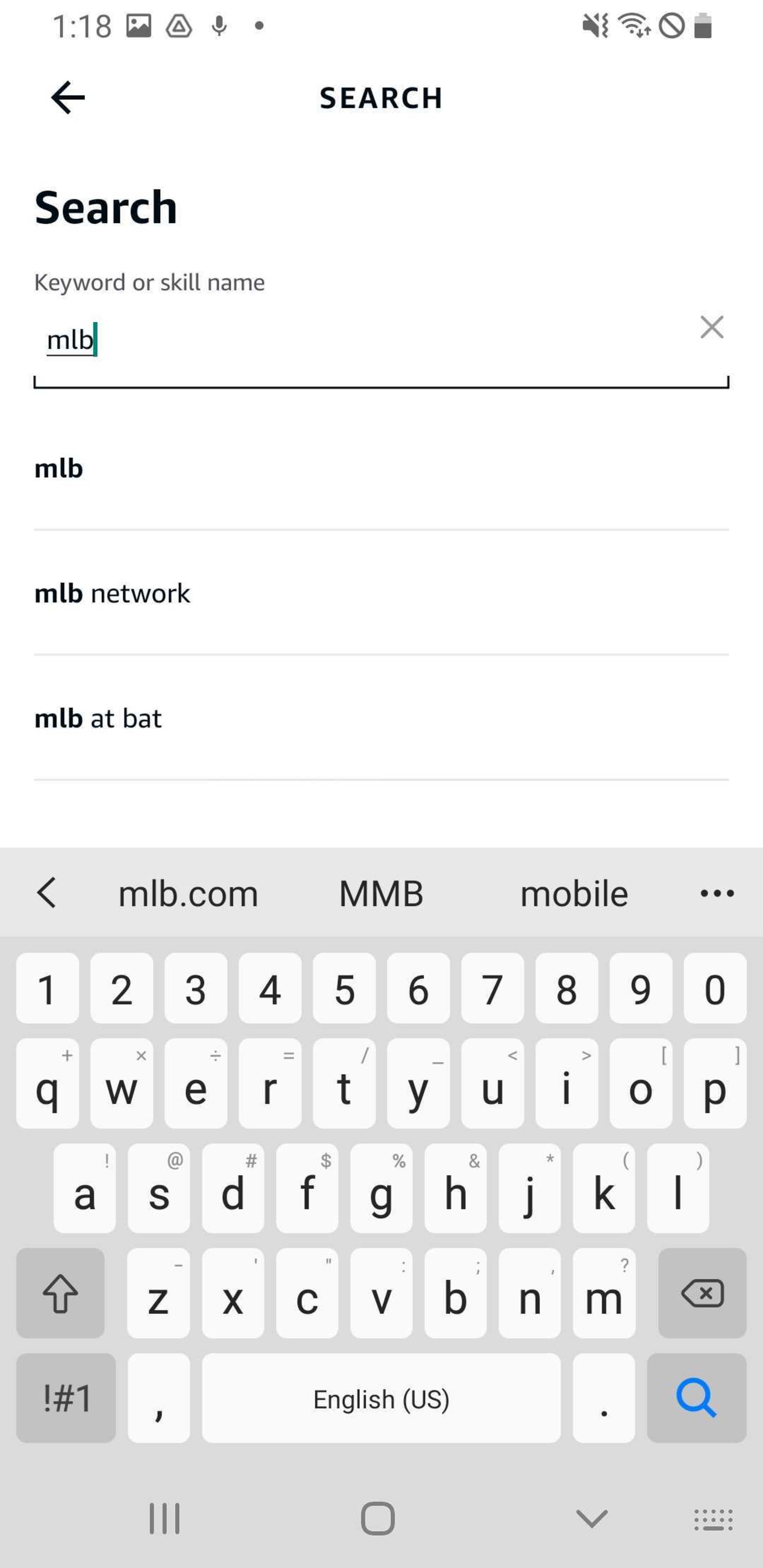This is a detailed descriptive caption for the image:

The screenshot depicts a mobile device's search page interface. At the very top of the screen is a white search bar. The black text within the search bar includes a back arrow icon on the left. Directly underneath, a larger text reads "Search" on the left side of the screen. Below this, smaller text prompts the user to "Enter keyword or skill name" above a text input field. The field currently has "MLB" typed in, with a small 'X' icon on the right side, providing an option to clear the text.

Beneath the text field are three suggested searches: "MLB," "MLB Network," and "MLB At Bat," each separated by a line divider. At the bottom of the screen, the device's keyboard is visible. The keyboard features predictive text options at the top, displaying suggestions such as "MLB.com," "MLB at Mobile," and another term next to an icon of three vertical dots. The main body of the keyboard follows, illustrating the standard layout of keys.